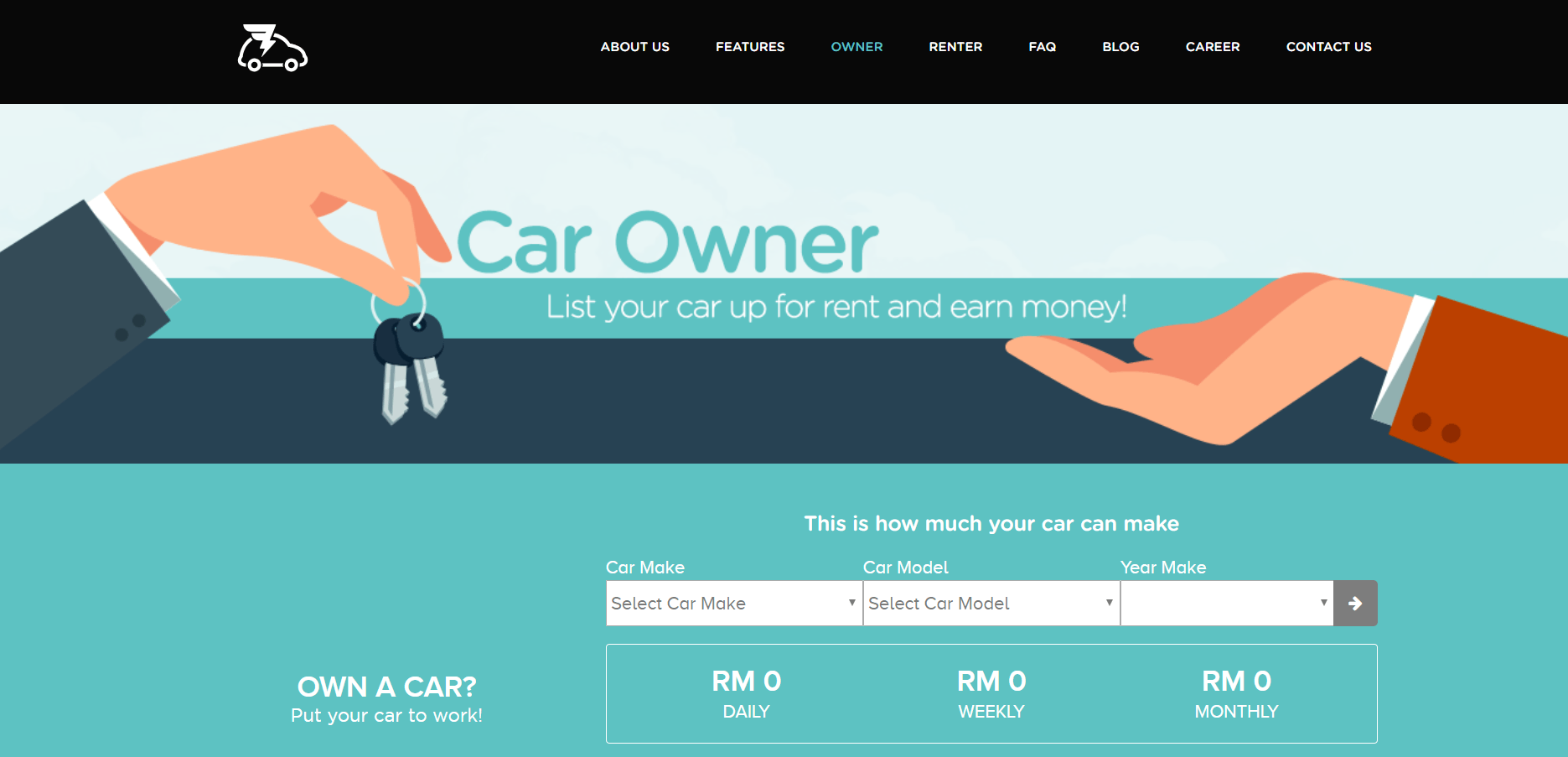In the image, the top features a black rectangle with a car picture displaying a flag-like element. Below, there are words in white, with one prominently in blue, followed by more white text. Beneath the black section is a gradient rectangle transitioning from light green to light blue, and then to a darker blue. The text "Car Owner" appears in this area. 

On the left side, an arm in a suit jacket and shirt extends, holding a pair of keys. Adjacent to this, another darker blue rectangle contains the phrase "List your car up for rent and earn money," and shows another arm, dressed in a white shirt and brown jacket, holding a cupped hand as if to receive something. 

Further below, another darker blue rectangle overlaps with a lighter blue section that reads, "Own a car?" followed by more text that is unclear. The statement, "This is how much your car can make," is visible. The car's make, model, and year are noted in a white rectangle with grey text, separated by grey lines and a dot at the end. Lastly, a grey square with an arrow pointing right, outlined in white, contains the text "RM0 daily," "RM0 weekly," and "RM0 monthly."